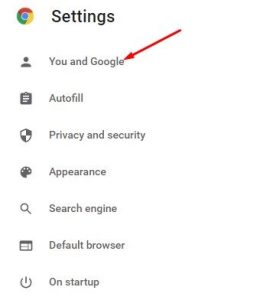The image is a detailed screenshot of the settings menu in Google Chrome, identified by its distinctive circular Chrome icon containing a central blue circle surrounded by three equal segments in red, green, and yellow. Positioned next to the Chrome icon, the word "Settings" is displayed in a semi-bold black font.

Below the "Settings" heading, the menu is divided into several distinct options, each accompanied by an icon on the left side:
1. **You and Google** - Represented by a minimalist gray icon depicting a person, consisting of a circle for the head and an oblong shape for the chest and shoulders.
2. **Autofill** - Illustrated with a gray clipboard icon.
3. **Privacy and Security** - Indicated by a shield icon that alternates between gray and white sections.
4. **Appearance** - Shown with a gray and white artist's palette icon featuring four circles.
5. **Search Engine** - Represented by a gray magnifying glass.
6. **Default Browser** - Depicted with a gray and white rectangle.
7. **On Startup** - Illustrated by a gray power button icon, which is a complete circle interrupted by a vertical gray line.

This menu provides a comprehensive overview of customization and security options available to users, each clearly identifiable by its respective icon.